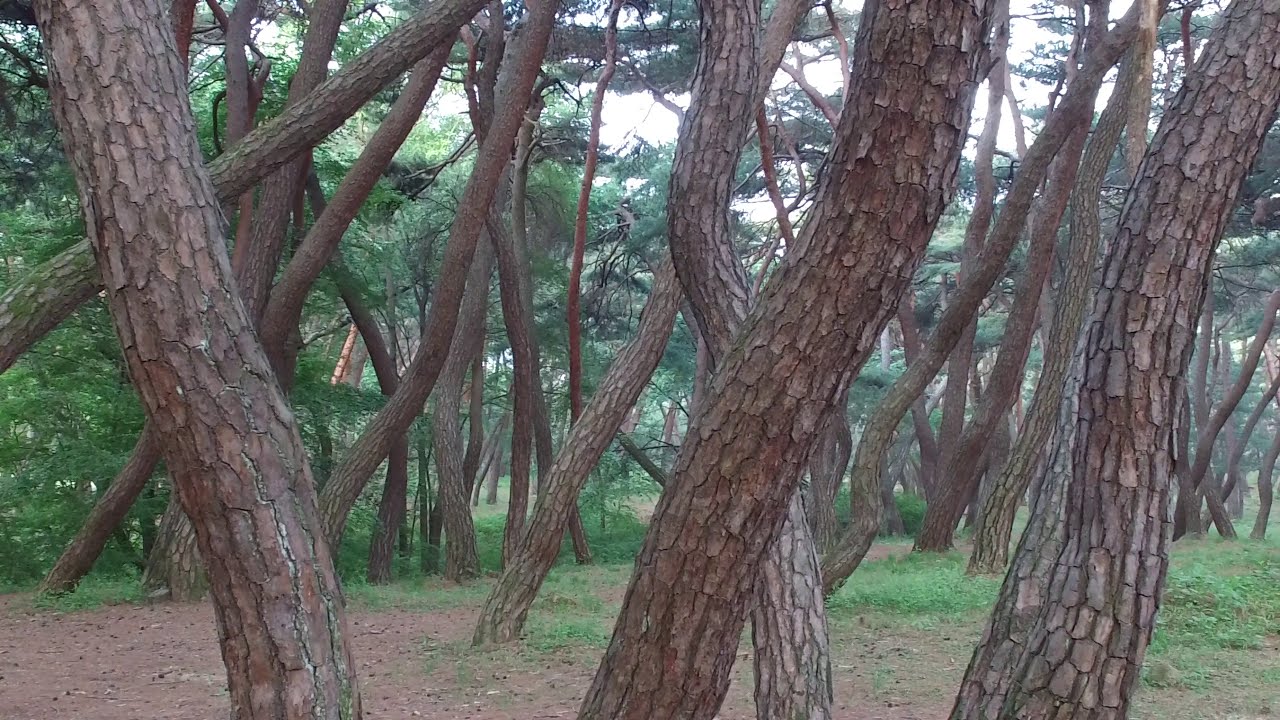This photograph captures a high-angle view of a dense forest where numerous tree trunks, adorned with rough, scaly brown bark, dominate the foreground. These trunks are intriguing as they grow in various unusual directions, with many slanting either to the right or left, and some even curving and twisting as they ascend from the brown and green ground. The forest floor mostly consists of dirt interspersed with patches of sparse grass. The image, possibly taken in the early morning due to the dim light and a faint glint of sunlight on one tree trunk in the background, reveals a clearing with more trees displaying lush green foliage. The scene is almost surreal, reminiscent of a painting, with the angled, sinuous trunks creating a striking visual contrast against the backdrop of coniferous trees cloaked in deep green leaves.